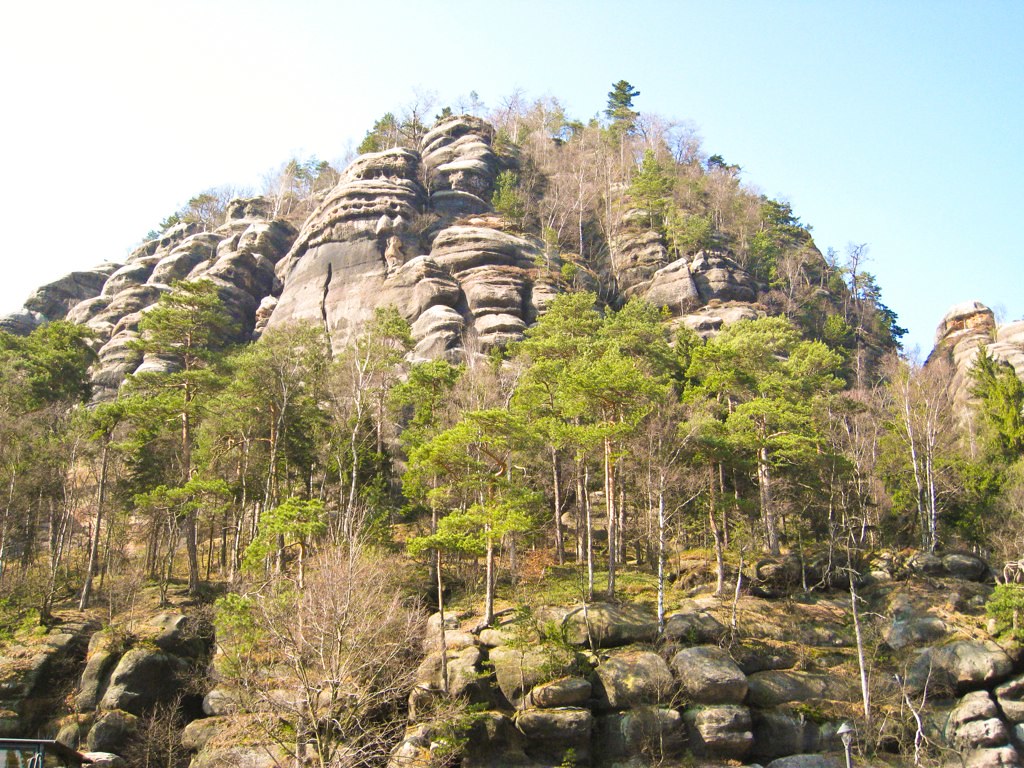The image captures a vast, rocky hillside with blocky, weathered boulders stacked upon one another, creating a rugged terrain that ascends steeply and rounds off at the summit. The rocks vary in color from light sand hues to areas adorned with moss, particularly underneath the sparse foliage and barren bushes that line the hillside. Numerous thin-trunked trees, some bare at the base, extend all the way to the top, their green canopies contrasting sharply against a sky that transitions from a bright white haze on the left to a rich turquoise on the upper right. The intricate layering, broken areas, and prominent fissures in the rocks make the scene particularly appealing for climbers. Amidst the greenery and dirt-filled expanse, the sunlight illuminates the upper sections of the rocks, indicating a lively yet challenging landscape that hints at years of natural weathering.